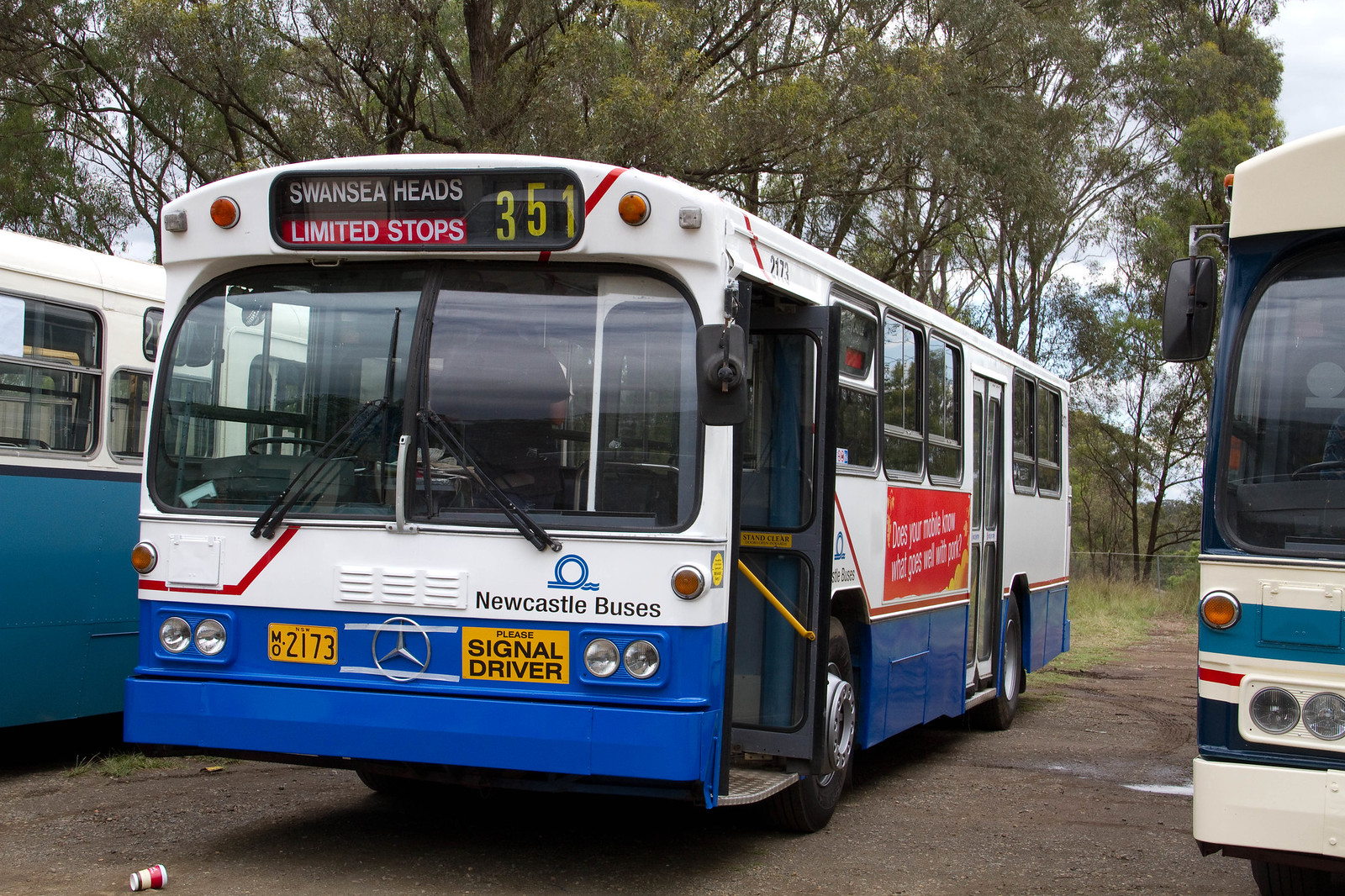This outdoor photograph features a prominently parked blue and white bus set against a backdrop of lightly vegetated brown gravel and tall, thin trees reaching into a partly cloudy blue sky. The central bus, more vividly detailed than the partial ones flanking it, showcases its distinct blue lower half up to the top of the tires and predominantly white middle and upper sections. Through the large front windshield, the bus driver is visible standing up. The bus's route information is prominently displayed, with "Swansea Heads, limited stops, 351" where the bus number, 351, is highlighted in gold. Just under the expansive windshield with large wipers, a sign reads "Newcastle Buses," while another sign on the blue section advises passengers to "please signal the driver." The front entrance of the bus is open while the rear remains closed. In front of the bus, a discarded white cup with a red stripe lies on the ground, adding a small touch of imperfection to the otherwise orderly scene.